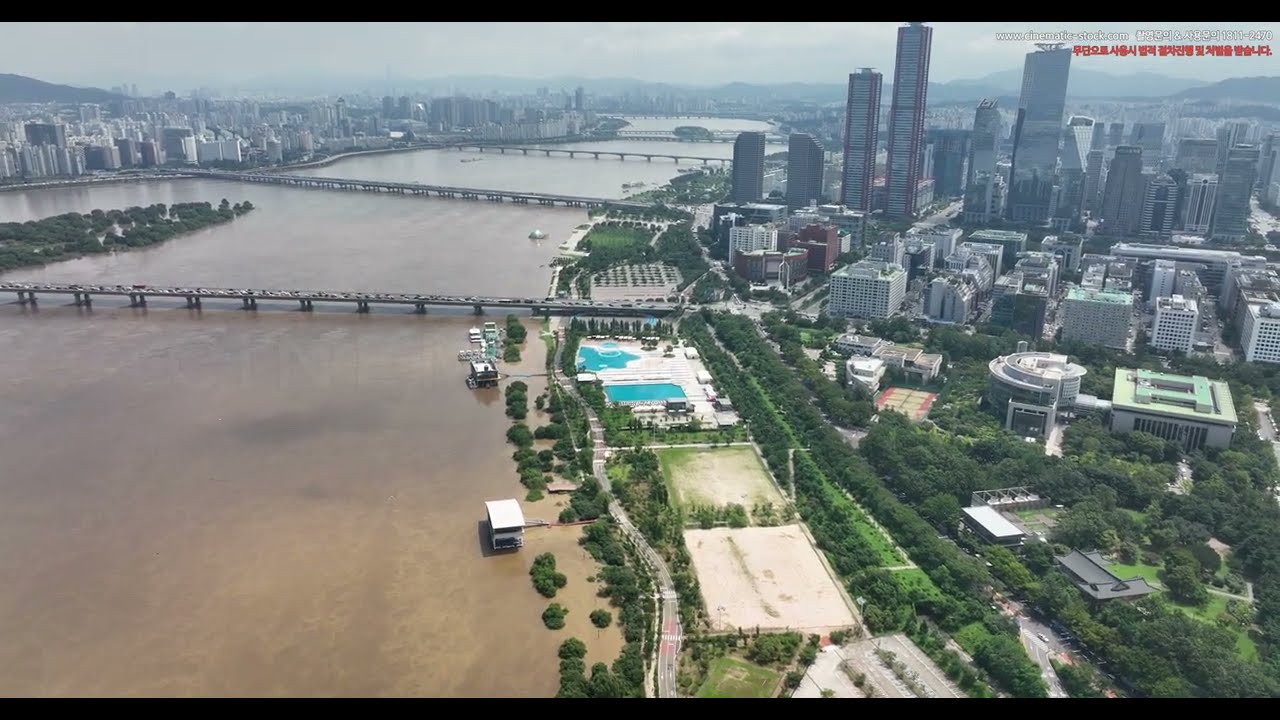This detailed aerial view of a sprawling urban landscape showcases a city bisected by a wide river, prominently featured on the left side of the image. The river, running from the bottom and curving gently to the right before bending back to the left at the upper part of the image, is spanned by three bridges: one positioned above the center and two more further up. The upper left-hand quadrant reveals a densely packed cluster of buildings, potentially apartments and offices, firmly abutting the river's edge, indicative of a bustling metropolis. The right bank mirrors the urban density with numerous tall buildings, interspersed with green spaces, possibly parks, creating a visually striking contrast. The bottom right section is lush with trees, which might belong to a significant park, adjacent to which are cement areas, including something blue resembling a pool or similar facility. Small boats dot the river, enhancing the sense of an active waterway. The muted, overcast ambiance adds depth to the scene, alluding to a day shrouded in clouds. In the top right corner, there are some Chinese characters alongside a watermark bearing "www.cinematicstock.com," suggesting an Asian locale, potentially confirmed by distant mountains on the horizon.